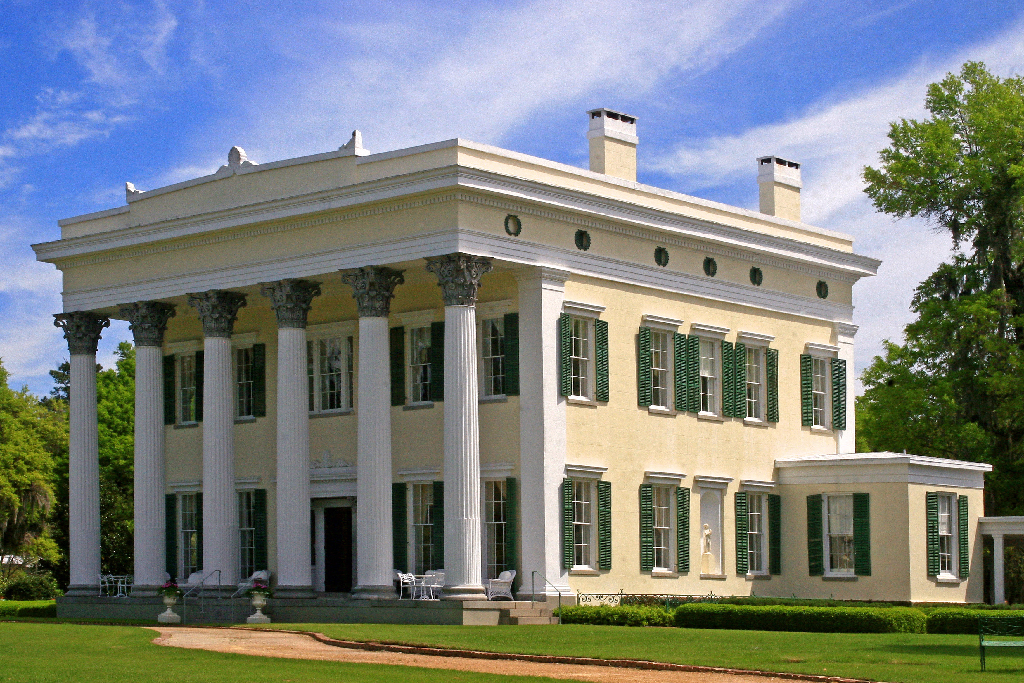The image showcases a large, ornate mansion characterized by its yellow-tan exterior and array of windows, each adorned with dark green shutters. The mansion stands two stories tall and features a grand front porch supported by six stately white columns, capped with dark gray at the tops. The porch is furnished with white chairs and possibly a white table. The building is complemented by a well-manicured, lush green lawn and a brick path leading up to it. Blue skies with scattered clouds form a picturesque backdrop, with trees and bushes framing the scene. Additionally, a small, single-story addition with two windows and green shutters extends from the main structure, suggesting a later expansion of the house. The roof is trimmed in white and includes two smokestacks.